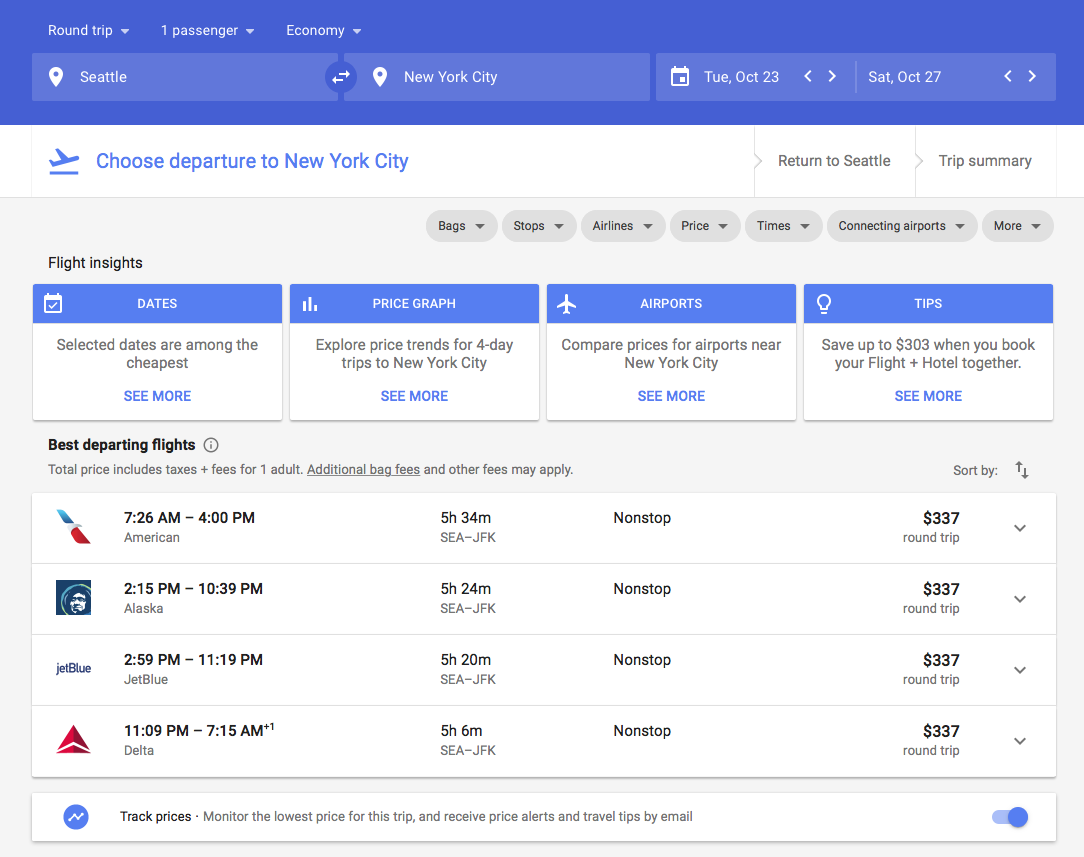In the image, the topmost section features a prominent blue bar indicating travel details: "Round-trip, one passenger, economy," with the rest of the bar left blank. Directly below, two lighter blue bars appear side-by-side, each with a location icon. The first bar displays "Seattle" and the second shows "New York City," with additional text reading "Round-trip." The trip dates are specified as departing on Tuesday, October 23rd, and returning on Saturday, October 27th. 

Beneath these bars, on a white background, is an icon of an airplane accompanied by the text "Choose departure to New York City." Below this, there are two options: "Return to Seattle" and "Trip Summary." Further down, seven small rounded rectangles provide filters or categories to refine the flight search: "Bags," "Stops," "Airlines," "Price," "Times," "Connecting Airports," and "More."

The next section appears as a graph, with columns labeled "Dates," "Price Graph," "Airports," and "Tips." Occupying nearly the bottom half of the screen, there's a section labeled "Best Departing Flights," which lists times, durations, whether the flights are non-stop, and their prices. At the very bottom, there's a notification option titled "Track Prices." This feature is currently activated, allowing users to monitor the lowest prices for this trip and receive price alerts and travel tips via email.